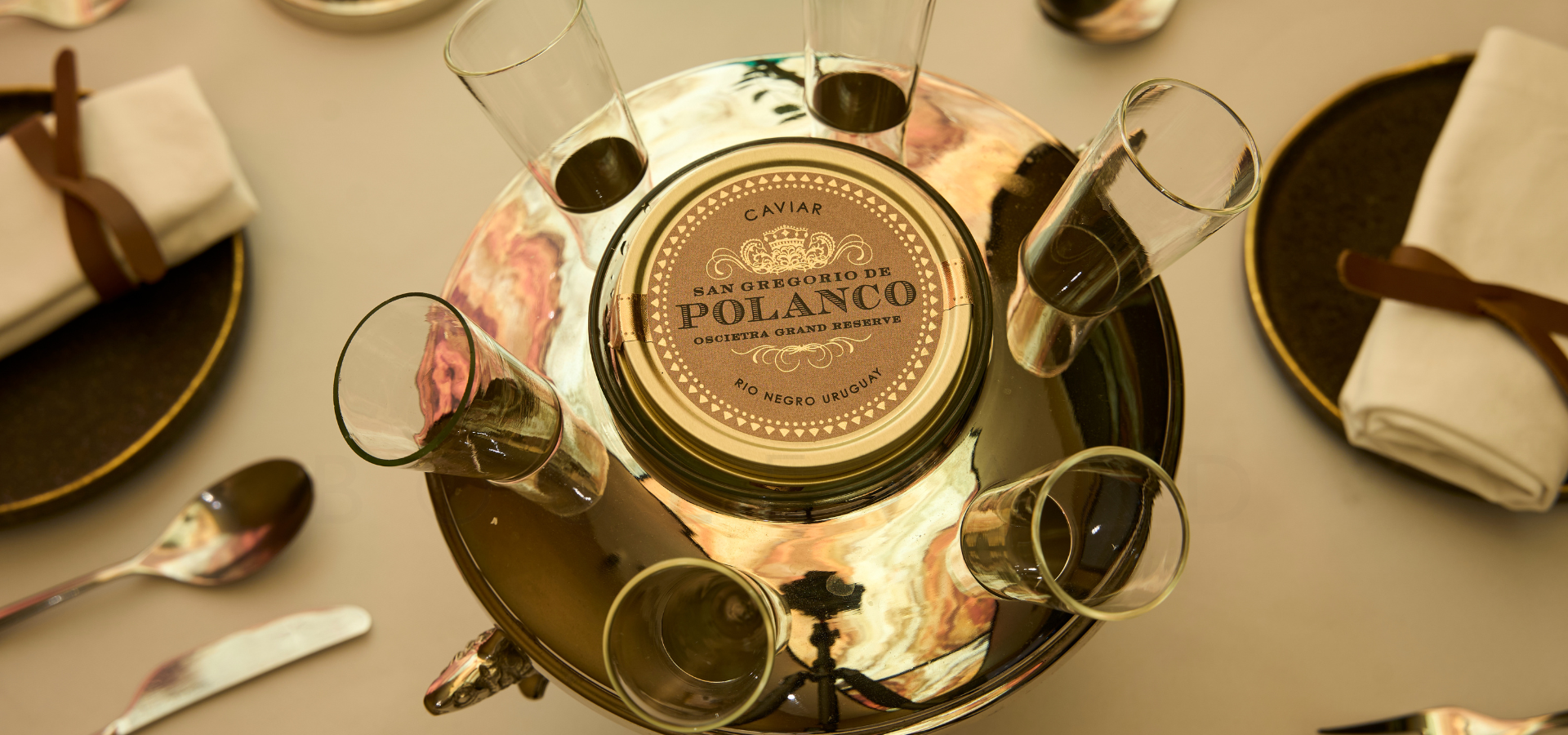This is a color photograph taken from above, showcasing an elegantly set dining table adorned with a light beige tablecloth. The focal point of the image is a luxurious golden container prominently placed at the center, engraved with the label "Caviar, San Gregorio de Polanco." The golden cylindrical vessel features six equally spaced cutouts, each holding a shot glass nestled within what appears to be an ice bucket, likely for chilling vodka to accompany the caviar.

Surrounding the central container are neatly arranged place settings. Each setting includes a plate topped with a white cloth napkin tied with a rustic brown leather strap, flanked by polished silverware comprising a spoon and a knife. The overall color palette of the image is dominated by warm, earthy tones, enhancing the sophisticated and cohesive atmosphere of the table setting.